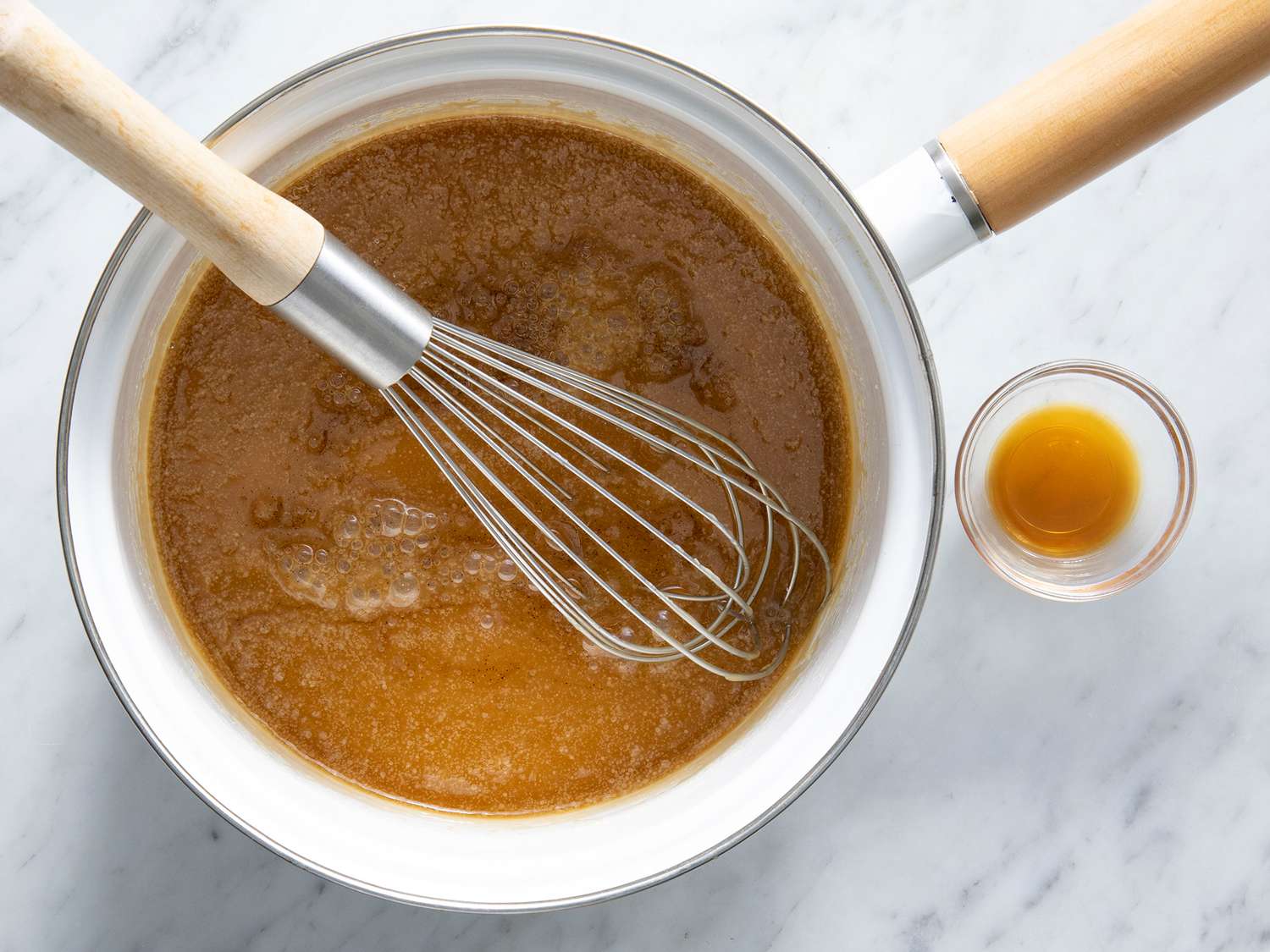A top-down photograph captures a white ceramic pot standing on a smooth marble countertop with faint black grains. The pot has a light brown wooden handle extending from the top left corner. Inside the pot, a shiny metallic whisk with a wooden handle is immersed in a caramel-colored, bubbly liquid. Positioned at the bottom right of the pot, the whisk appears clean, suggesting minimal activity. The liquid inside the pot resembles caramelizing sugar or possibly brown butter, characterized by its rich amber tones and slight bubbling. To the right of the pot is a small, clear glass beaker containing a similar amber liquid, though it appears clearer and less mixed. The marble countertop and the general kitchen setup suggest preparations for a cooking or baking activity involving caramel or melted sugar.